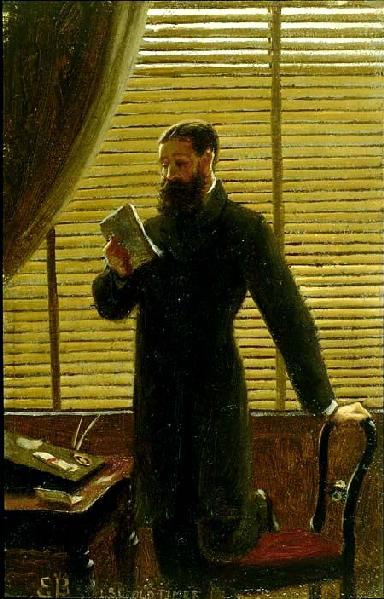This vertical, rectangular painting depicts a man from an earlier era standing near a small brown wooden desk. He is positioned with his left knee resting on a black wooden chair with an open, rounded back and a plush red velvet cushion. The man, who has short dark hair and a full, bushy black beard, is dressed in a dark, nearly black suit, with a white undershirt visible at his collar and wrists. He is wearing matching pants and glasses. In his right hand, he holds a small book or notebook, and he is looking down at it intently. His left hand grips the top of the chair for support. The scene is set before a large window covered with white and wood blinds and complemented by a flowing, tied-back dark brown curtain. The background features yellow and brown hues with hints of green, creating a warm ambiance. Papers and possibly a feather pen lie on the small desk in front of the man, which also holds a black slanted writing board.